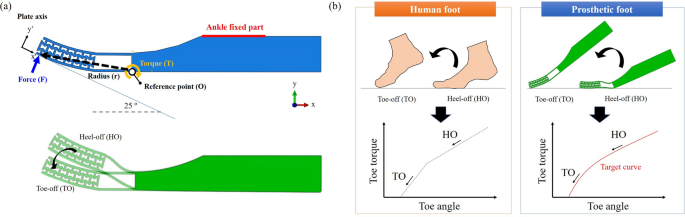The image is a horizontal rectangular diagram that compares the movement of a human foot and a prosthetic foot. The left-hand side, labeled 'A,' features two diagrams depicting a foot in motion, with annotations like "ankle fixed part," "torque," "radius," and "force." The top diagram has a blue block with a curved area to its left, demonstrating foot motion; the bottom diagram is similar but shorter and highlighted in green, with a focus on "toe off." 

On the right-hand side, labeled 'B,' are diagrams comparing a human foot and a prosthetic foot. The human foot is displayed on an orange strip and is shown rising onto the toes, with annotations for "toe off" and "heel off." Below this is a line graph tracking "toe torque" and "toe angle."

Adjacent to it, the prosthetic foot is presented on a blue strip, marked in bright green, with similar "toe off" and "heel off" points. It also includes a green rectangle representing the prosthetic movement, with an accompanying chart illustrating "toe torque" and "toe angle." A line labeled "target curve" is present on the prosthetic foot chart, underscoring the comparison between natural and artificial foot motion.